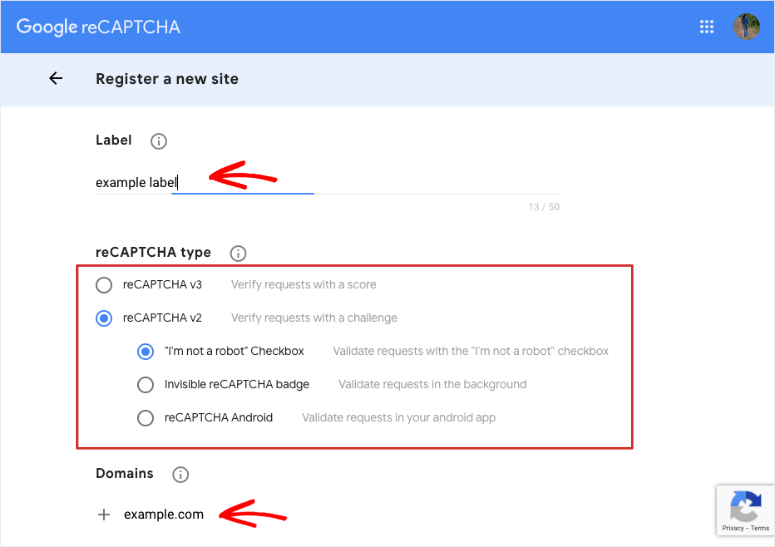This is a screenshot of a web page oriented in landscape, bordered by a thin gray line on three sides: bottom, left, and right. The top of the image features a light blue, horizontal header with white text in the top left corner reading "Google reCAPTCHA". Adjacent to this text, towards the right, is a 3x3 grid of dots and an avatar in a circular frame depicting a person standing in nature.

Below the header is a gray horizontal bar, featuring a left-facing arrow followed by the text "Register a new site". 

The main body of the screenshot consists of a white, landscape-oriented rectangular section. At the top of this section, "Label" is written in black font, with "example label" written directly beneath it. This section has a thin gray border below the text and a small blue line highlight next to "Label". A red, hand-drawn arrow is pointing to the word "Label".

Further down, there is a heading titled "reCAPTCHA type" accompanied by a long, rectangular red box containing multiple radio button options. The options include "CAPTCHA version 3" and "CAPTCHA version 2", with the latter selected and highlighted in blue. The selected option reads "I am not a robot check box".

At the bottom of this section, another red arrow points to the text "example.com".

This detailed description provides a clear visualization of the web page layout, emphasizing the elements related to Google's reCAPTCHA configuration.